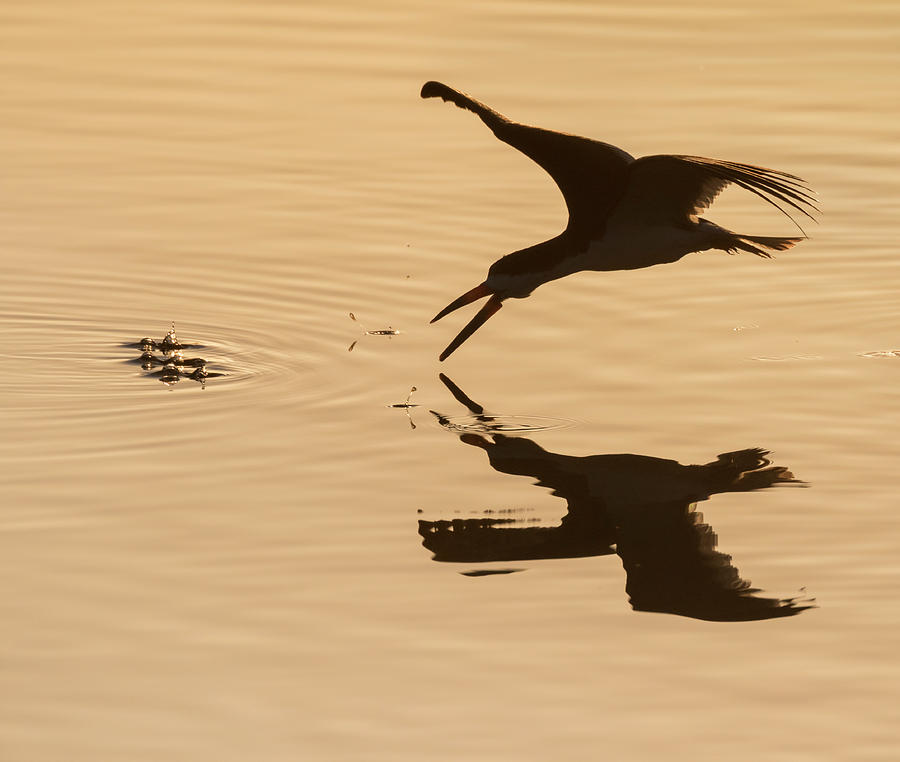In this captivating image taken at either dusk or dawn, a dark, large bird, possibly a seagull, is captured in mid-flight just one foot above the water. With its beak open, the bird appears to be in hunting mode, aiming to snatch a fish from the water below. The lighting creates a dramatic silhouette effect, accentuating the bird's black outline and long, narrow beak. The water beneath reflects the bird's silhouette, adding a sense of symmetry to the scene. The water has an orangey-brown hue, likely due to the sun's position at the horizon. To the left of the bird, the water ripples, possibly indicating the presence of small fish or seaweed that has caught the bird's attention. This serene yet dynamic moment is bathed in warm hues of brown and orange, suggesting the photograph captures the ethereal beauty of sunset.